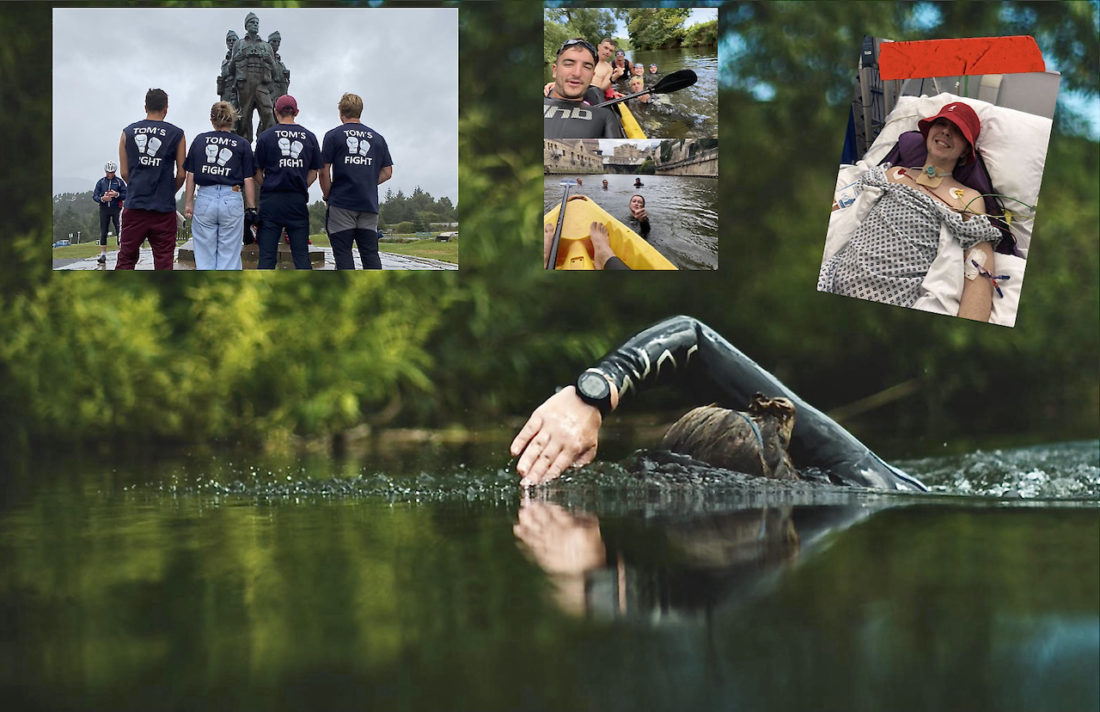The main photograph depicts a Caucasian woman swimming in a calm, greenish body of water, likely a lake, with her arm outstretched in a breaststroke. She wears a diver's watch and is swimming towards a blurred background filled with trees and bright green foliage. Overlaying this main image are three smaller photographs at the top. The top left photo shows five individuals standing with their backs to the camera, all wearing shirts that say "Tom's Fight," facing a statue of soldiers which appears to have a World War II theme. The top middle photo captures a group of people, both men and women with varying hair colors, kayaking together in a yellow canoe on the same greenish water, with additional people swimming behind them. The top right photo portrays a young girl with a red hat, lying in a hospital bed connected to various monitors, possibly part of a tribute to her as Tom.